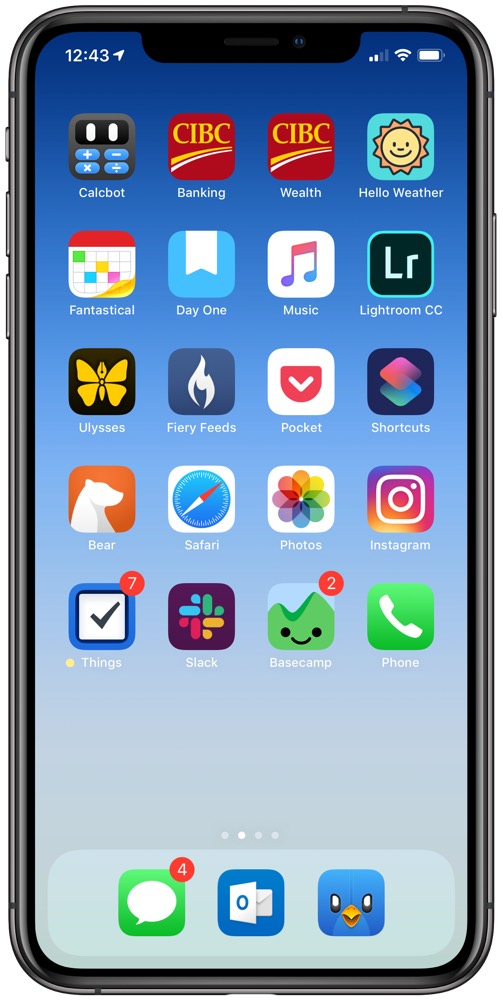Detailed caption: 

This image is a screenshot of a smartphone. The device itself has a medium gray border featuring three buttons on the left side and one button on the right. The screen displays a gradient blue background that transitions from dark blue at the top to almost white at the very bottom. The status bar at the top shows the time as 12:43, along with internet and battery charge icons.

Beneath the status bar, the home screen is organized into five rows of app icons, followed by a dock containing three frequently used apps. 

- **First Row:**
  - *Calcbot*: An app with a black background featuring two white bars resembling robot eyes and symbols for addition, subtraction, multiplication, and division.
  - *CIBC Banking*: A red icon labeled "CIBC" with the word "banking" below it.
  - *CIBC Wealth*: Another red icon labeled "CIBC" with the word "wealth" beneath it.
  - *Hello Weather*: This app icon has a blue background with an animated smiling sun.

- **Second Row:**
  - *Fantastical*: A calendar app with this title under the icon.
  - *Day One*: Featuring a blue background with a bookmark image.
  - *Music*: An icon with a musical note and the word "music" beneath it.
  - *Lightroom CC*: Displaying a black background with the letters "LR" on it.

- **Third Row:**
  - *Ulysses*: An app with a black background and a yellow butterfly, labeled "Ulysses."
  - *Fiery Feeds*: Featuring a dark purple/navy background with a flame icon, labeled "Fiery Feeds."
  - *Pocket*: Displaying a white background with a red pocket and a white "V," labeled "Pocket."
  - *Shortcuts*: An icon with a navy background and two squares (one pink, one blue), labeled "Shortcuts."

- **Fourth Row:**
  - *Bear*: An app with a silhouette of a bear on an orange background.
  - *Safari*: Displaying a white background with a compass icon.
  - *Photos*: Featuring a white background with a colorful, kaleidoscope-like image of a flower.
  - *Instagram*: An icon featuring a camera with a pink, orange, and blue gradient background.

- **Fifth Row:**
  - *Things*: Displaying a blue background with a white square containing a black checkmark, and a red circle with the number "7."
  - *Slack*: An app with a purple background and different colored bars.
  - *Basecamp*: Featuring an animated mountain icon with a red circle containing the number "2."
  - *Phone*: An icon with a green background and a phone symbol.

- **Dock:**
  - A green bubble with a talk icon showing four notifications in a red circle.
  - A blue mail icon.
  - A blue bird icon, likely representing Twitter, though it resembles an animated bird.